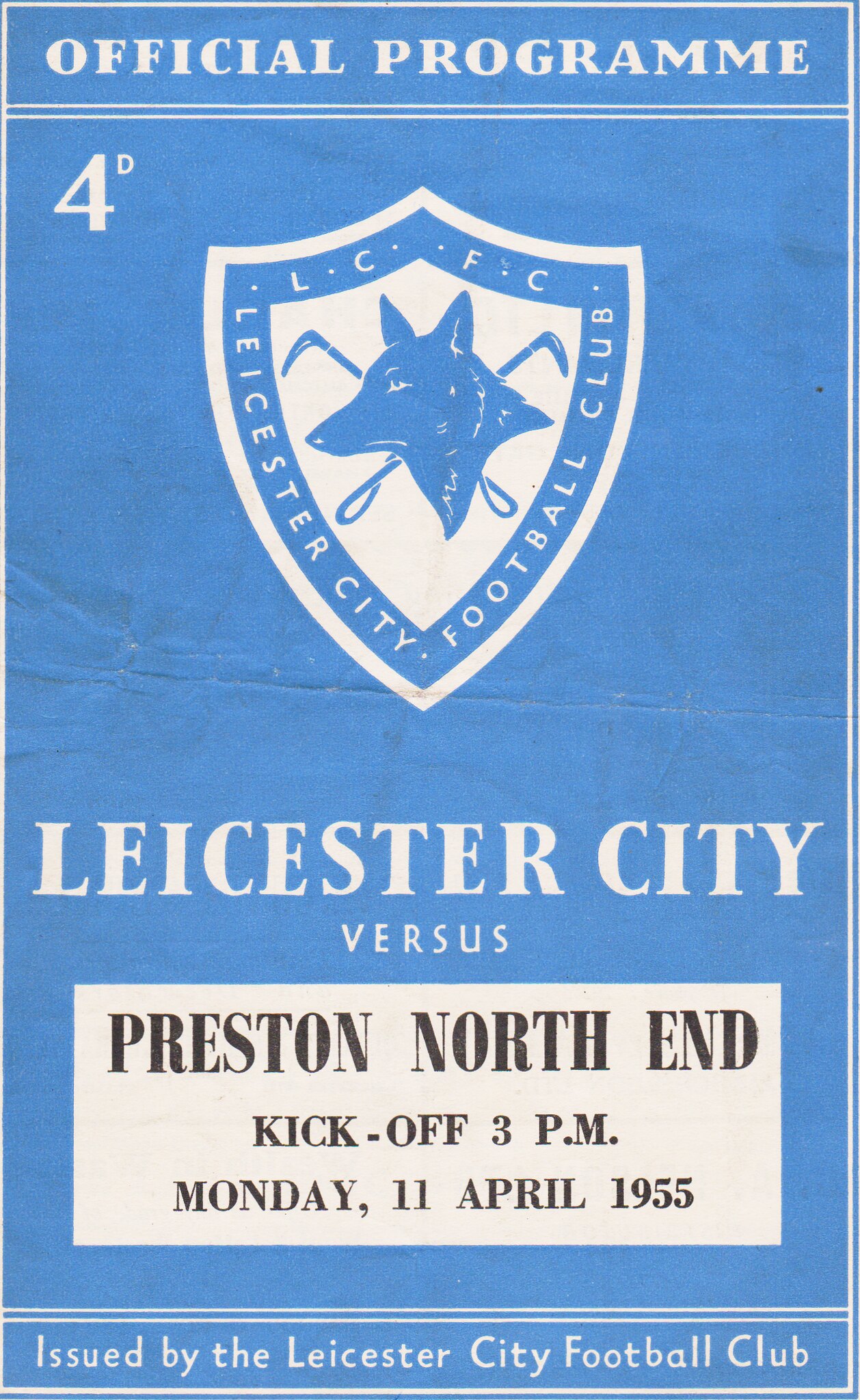The image is an official program for the football match between Leicester City and Preston North End, scheduled for 3 p.m. on Monday, April 11th, 1955. The background of the program cover is blue, featuring prominent text at the top that reads "Official Program" within a white rectangle. Below this text is a detailed logo resembling a shield with a wolf's head at its center, and the inscription "Leicester City Football Club." Additionally, there are some small details like what appear to be hockey sticks and loops just below the neck of the wolf. Further down the cover, the text "Leicester City versus Preston North End" is displayed, followed by the match details in black font within a white rectangle. At the very bottom, it states, "Issued by the Leicester City Football Club." The top left corner also features the price, marked as "4 D".